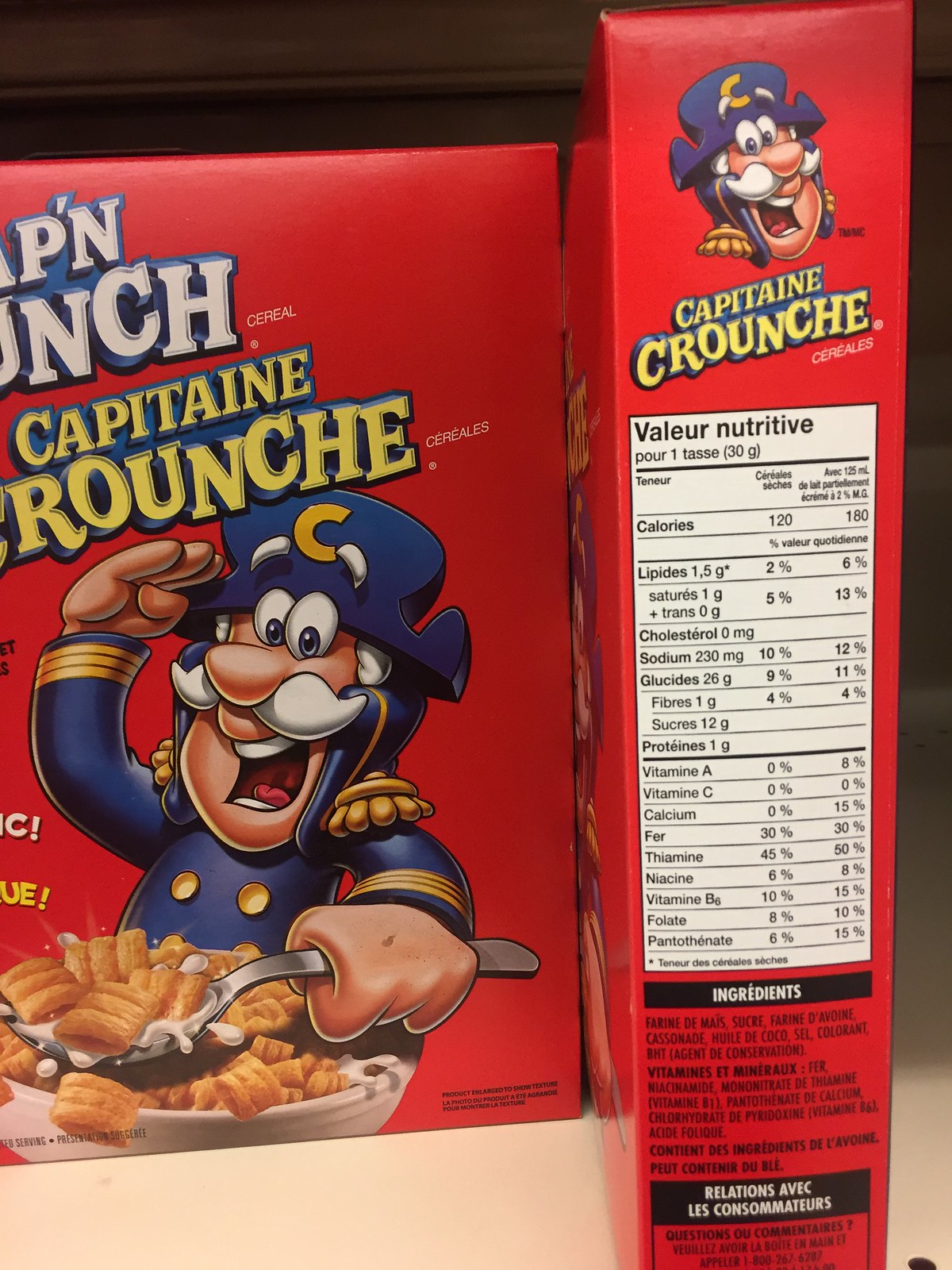This indoor, color photograph is a close-up image showcasing two boxes of Cap'n Crunch cereal, with a charming twist. Dominating the left of the frame, we see the front face of a Cap'n Crunch box, featuring a classic red background. The familiar cartoon image of Cap'n Crunch, in his iconic blue uniform, is central, with his right hand raised in a salute and his left hand dipping a spoon into a bowl of cereal. Below the illustration, the text reads "Cap'n Crunchay," indicating a French version of the beloved cereal.

To the right, the side panel of the same box is visible, displaying nutritional information in French. The white rectangular nutrition label at the top reads "Valeur Nutritive," which translates to "Nutritional Value." Detailed nutritional facts are listed, including 120 calories, 1.5 grams of lipids, 0 milligrams of cholesterol, 230 milligrams of sodium, 26 grams of sugar, and 1 gram of protein.

Both cereal boxes are sharply focused and positioned on a light tan shelf, highlighting the intriguing dual language packaging.